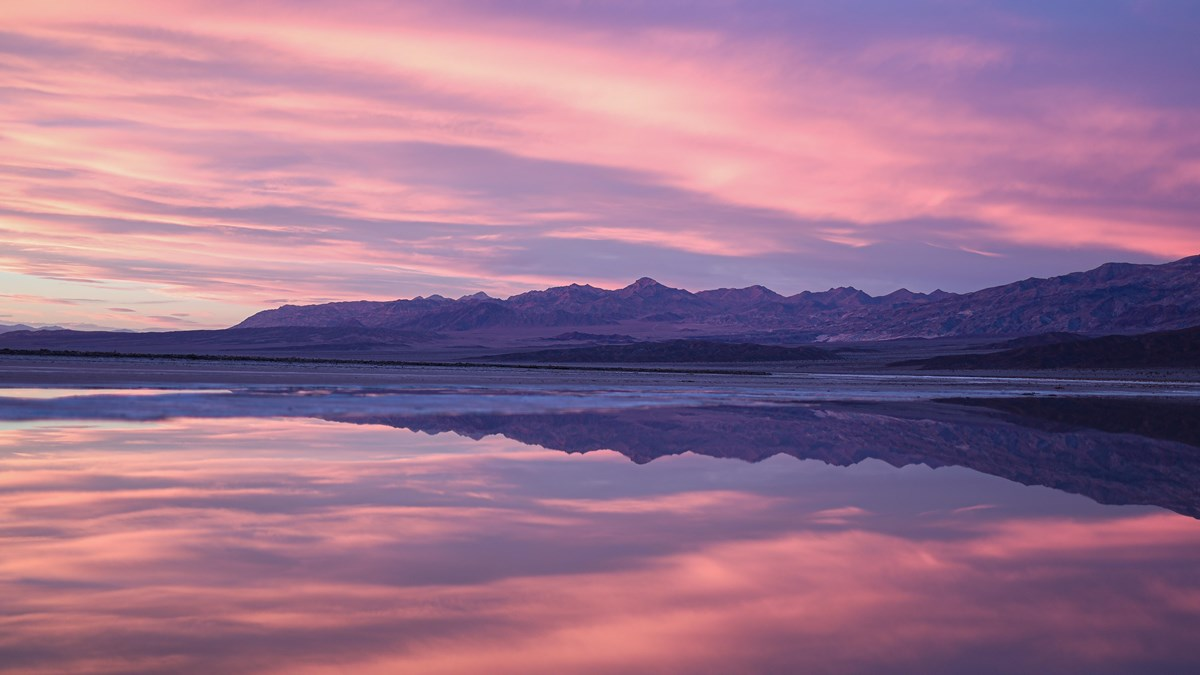This photograph captures a serene lake at either sunset or sunrise, with a tranquil, glass-like surface that perfectly mirrors the vibrant sky and the distant, low-lying mountains. The sky is a stunning tapestry of pink, purple, and red hues, with wispy clouds that are predominant, giving the scene a mystical, almost ethereal quality. The mountains, or perhaps hills, ascend slightly from the dark shoreline, adding depth and contrast to the landscape. Their rocky textures are faintly visible, hinting at a rugged terrain. The reflection on the lake doubles the beauty, showcasing the elegant streams of color and the layered cloud patterns. Despite the possible presence of settlements on the distant hills, they remain shrouded in twilight's mystery, blending into the scenic harmony of nature's palette.